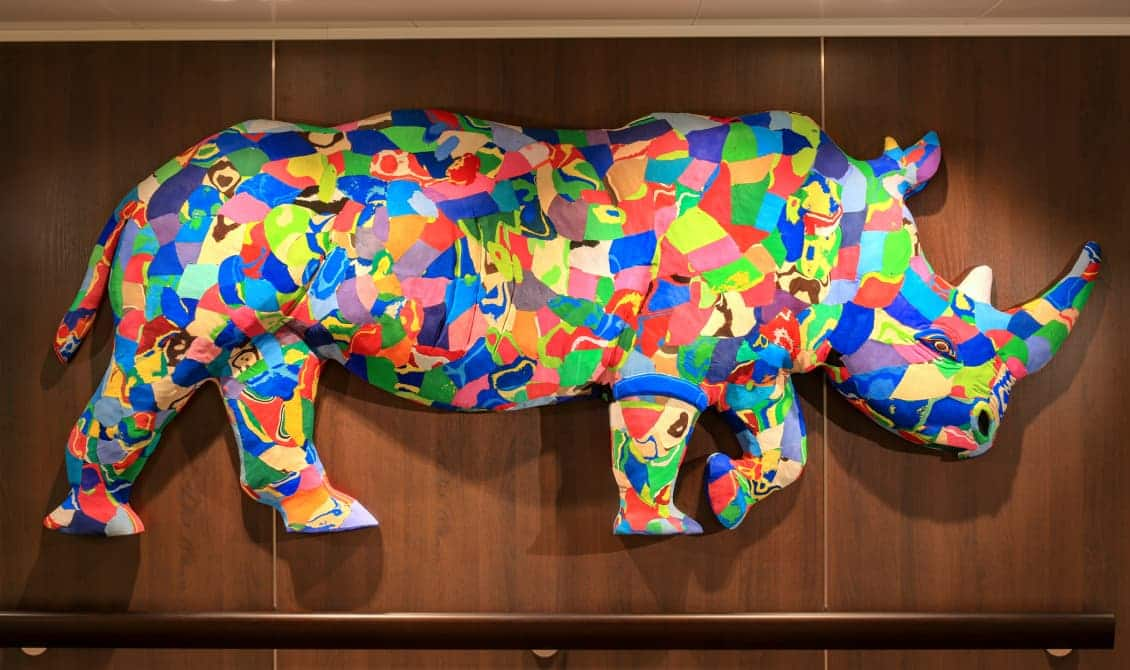This image captures a vibrant and artistic representation of a rhinoceros on display inside a museum. The 3D sculpture, mounted against a backdrop of brown wooden panels, features a kaleidoscope of colors including shades of blue, green, red, yellow, pink, orange, white, black, and brown. The rhino, portrayed in profile facing right, showcases intricate patterns of squares and rectangles across its surface, giving it an arresting multicolored appearance. Notably, it has two horns, with one distinctively white, and is shown walking, complete with four legs and a tail. Illuminated by artificial light that emphasizes its vivid colors, the artwork is positioned above a wooden handrail, adding a complementary earthy tone to the overall composition.